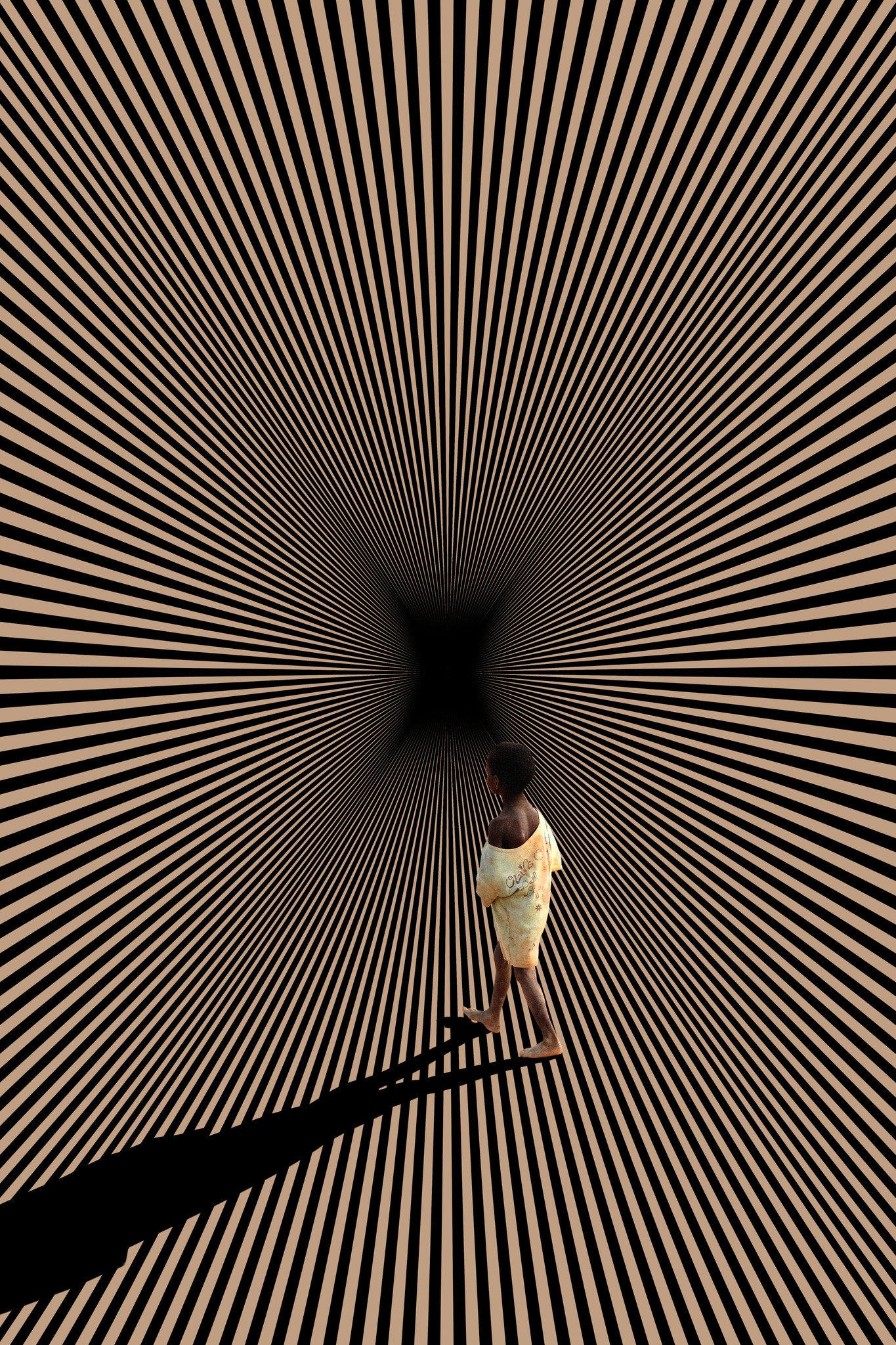The image depicts an African American child, barefoot and dressed in a long, oversized, yellow tie-dye shirt that resembles a dress, with the text "Ghania" on it. The child strides across a room designed to evoke a powerful optical illusion. The background features an intricate pattern of black and beige lines that converge into a central black square, creating a vortex-like effect that draws the viewer's eye to the middle. The lines give the impression of peering into a deep pit or void. The child’s shadow stretches long to the left, contributing to the surreal and illusionary quality of the scene. The setting remains ambiguous, adding to the overall mysterious and intriguing nature of the image.